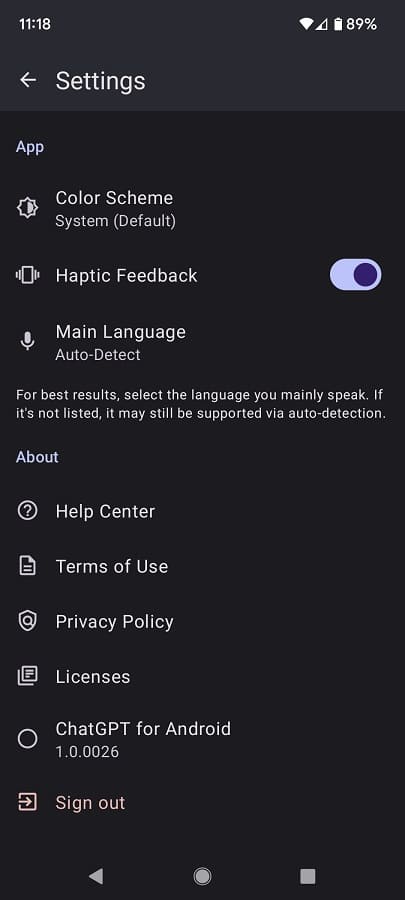This is a detailed description of the settings panel for the ChatGPT for Android app. 

At the top of the interface, the panel is labeled "Settings." Above this, the status bar displays the current time as 11:18, with the phone’s battery level at 89%. 

Directly under the "Settings" label, the "App Settings" section begins. The first setting listed is "Color Scheme," which is currently set to "System Default." Options available for the color scheme include "Dark," "Light," and "System Default." 

Following the color scheme setting, there is the "Haptic Feedback" option, allowing users to enable or disable haptic feedback, which is typically used for key presses during text input.

Next, the "Main Language" setting is displayed, with "Auto Detect" activated. This setting automatically detects the language based on the user’s country. There is a message advising users to select the language they primarily speak for the best experience. If the specific language is not listed, it may still be supported through auto detection.

Below the language setting is the "About" section, containing links to the "Help Center," "Terms of Use," "Privacy Policy," "Licenses," and information about the app itself, listed as "ChatGPT for Android version 1.0.0026." 

Finally, at the bottom of the settings panel, there is an option to sign out of the app.